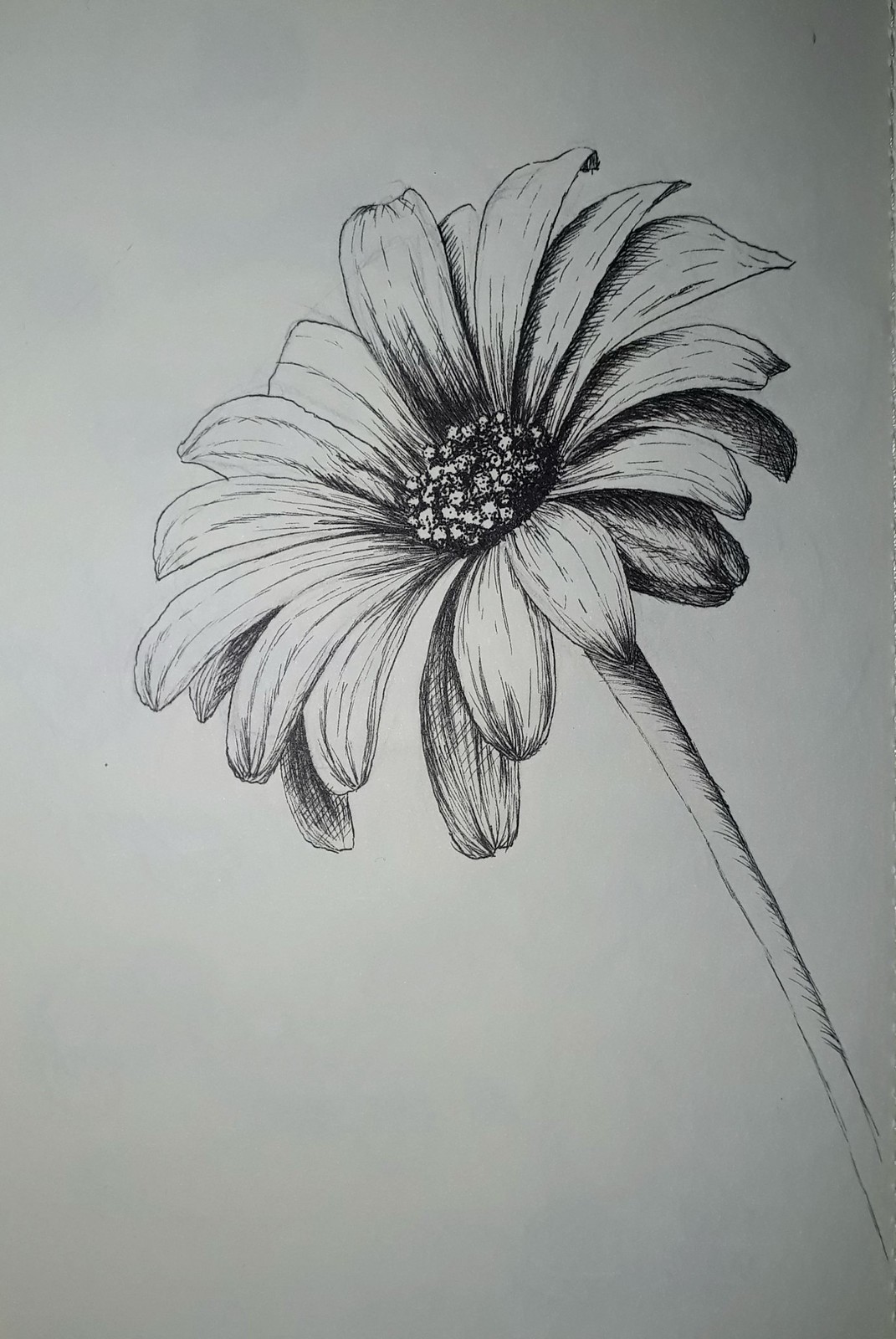This is a detailed image of a meticulously drawn flower on blank white notebook paper, depicted in black and white. The flower is oriented diagonally, with a thin, elongated stem extending from the lower right to the upper left. The drawing showcases a bloom with two layers of petals. The top layer has approximately 14 - 15 thin, medium-length petals, while the lower layer has fewer petals, each rendered with subtle shading to convey depth. The central receptacle reveals intricate reproductive parts composed of numerous small, circular structures. The stem and selected leaves feature shading on the right to accentuate shadows. The drawing is finely detailed, particularly at the tips of the petals. The surrounding paper is devoid of any text or signatures. Notably, the upper right corner displays part of the notebook’s wire binding. The overall image maintains clear focus, emphasizing the skill and detail in the pencil work.